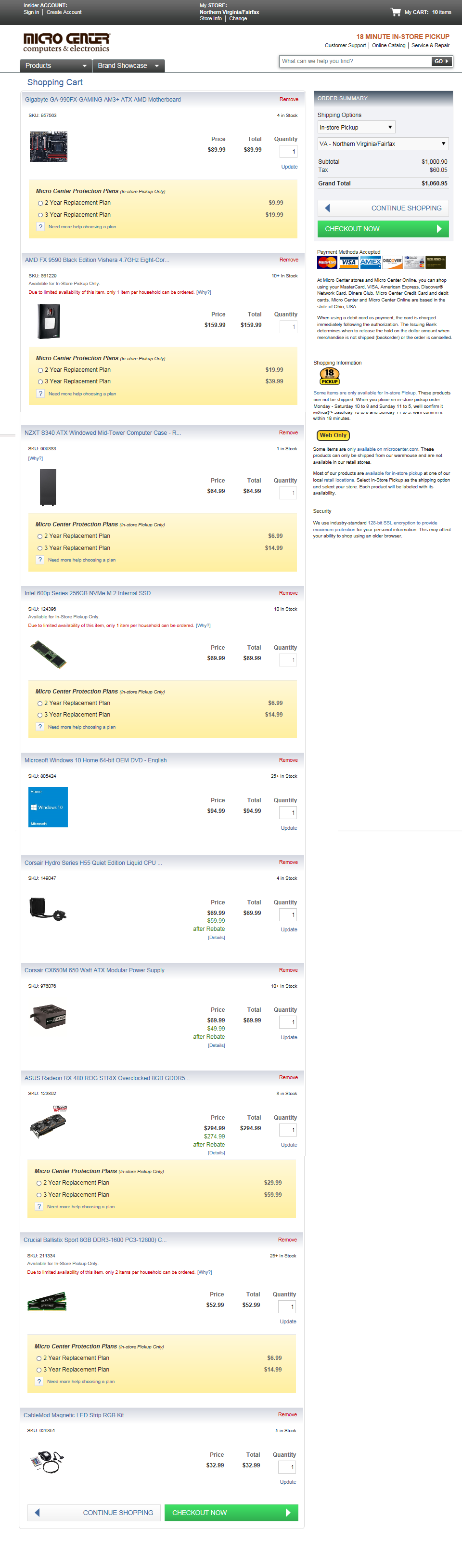This image captures a shopping cart from the Micro Center website, listing a variety of computer components and accessories along with their respective prices and quantities. The cart includes a Gigabyte Gaming Motherboard priced at $89.99, and an AMD FX Black Edition 4.7 GHz 8-Core Processor for $159.99. Additionally, there's an NZXT S340 ATX Windowed Mid-Tower Computer Case for $84.99 and an Intel 600 Series 256GB NVMe M.2 Internal SSD for $70.00.

Other items include Microsoft Windows 10 64-Bit OEM DVD in English for $94.99, a Corsair Hydro Series H55 Quiet Edition Liquid CPU Cooler for $89.99, and a Corsair CX650M 650W ATX Modular Power Supply at $69.99. The cart also features an Asus Radeon RX 480 ROG Strix Overclocked 8GB GDDR5 PCI Express 3.0 Graphics Card priced at $294.99, a Crucial Ballistix Sport 8GB DDR3-1600 PC3-12800 CL9 Dual Channel Desktop Memory Kit for $159.99, and a CableMod Magnetic LED RGB Kit for $39.99.

Optional protection plans for each item are available at additional costs. The subtotal before tax amounts to $1,050.00, with sales tax bringing the grand total to $1,061.45. The cart includes a total of 10 items, and offers options for in-store pickup and various payment methods including Visa, MasterCard, American Express, and Discover. Note that some items are web-only, and security measures for online transactions are indicated.